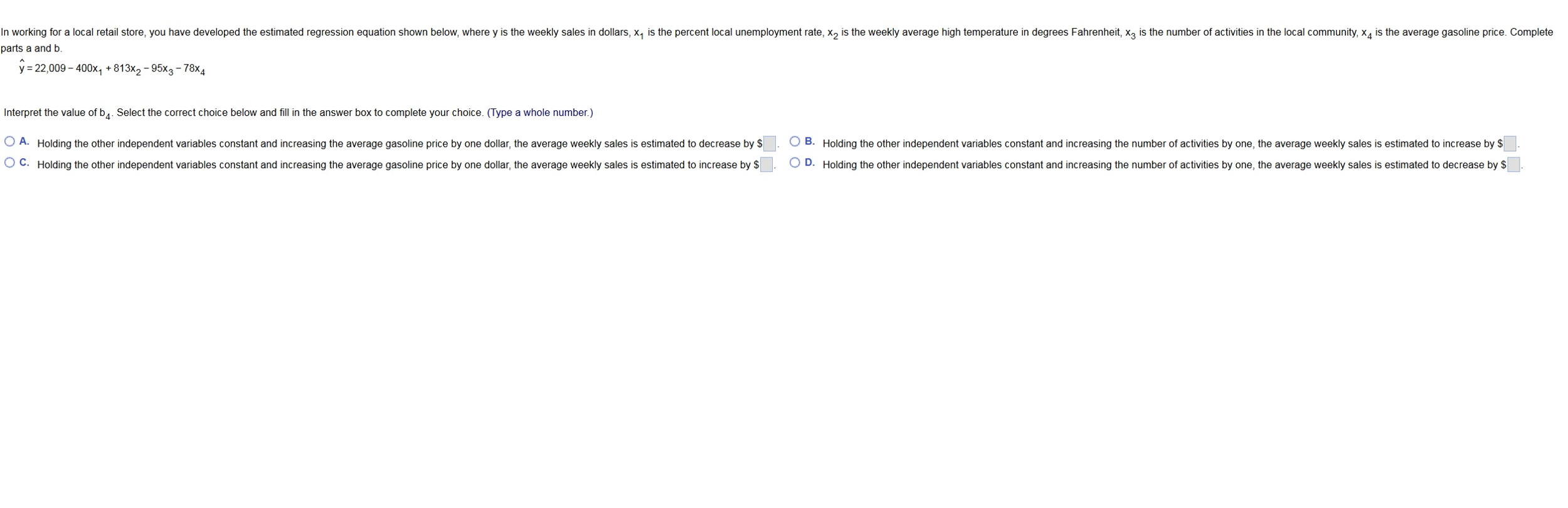Here's the cleaned-up and detailed caption for the image:

---

The image is a screenshot of a web page containing a problem related to regression analysis. The text is in small print and describes a scenario where one is working for a local retail store and has developed an estimated regression equation. The equation given is:

\[ \hat{Y} = 22,009 - 400X_1 + 813X_2 - 95X_3 - 78X_4 \]

In this context:
- \( Y \) represents the weekly sales in dollars.
- \( X_1 \) is the local unemployment rate (in percent).
- \( X_2 \) is the weekly average high temperature (in degrees Fahrenheit).
- \( X_3 \) is the number of activities in the local community.
- \( X_4 \) is the average gasoline price (in dollars).

The screenshot instructs to complete parts A and B of the problem. Part A involves interpreting the coefficient \( B_4 \). The questions posed are multiple-choice, with the choices:

**A.** Holding the other independent variables constant, and increasing the average gasoline price by one dollar, the average weekly sales is estimated to decrease by $_____ (a whole number to be filled in).

**B.** Holding the other independent variables constant, and increasing the number of activities by one, the average weekly sales is estimated to increase by $_____ (a whole number to be filled in).

**C.** Holding the other independent variables constant, and increasing the average gasoline price by one dollar, the weekly sales are estimated to increase by $_____ (a whole number to be filled in).

**D.** Holding the other independent variables constant, and increasing the number of activities by one, the average weekly sales are estimated to decrease by $_____ (a whole number to be filled in).

This problem requires selecting the correct choice and filling in the appropriate dollar amount based on the regression equation provided.

---